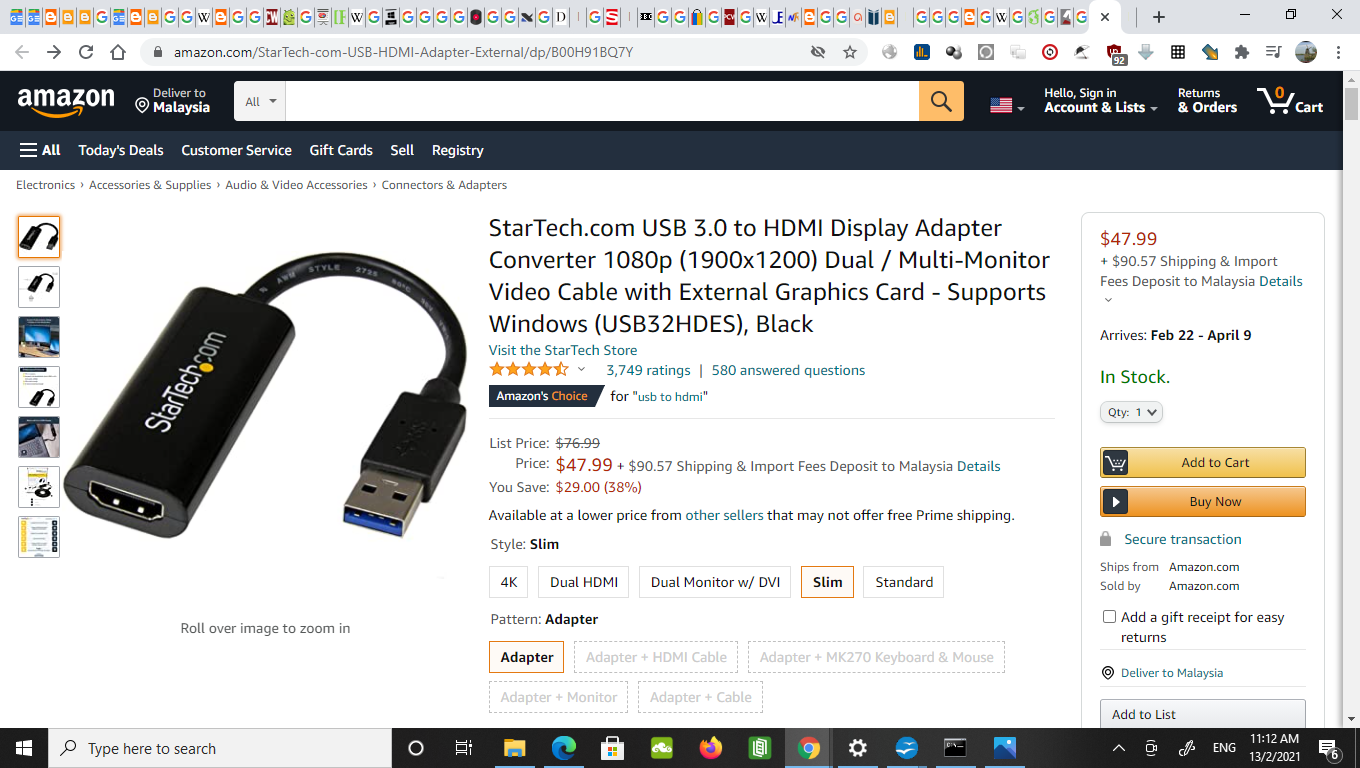The image portrays a computer screen with an extensive amount of browser tabs open, estimated between 40 to 50. The setup includes various Google Chrome tabs, some featuring Google Docs, and an older Internet Explorer window. On the right-hand side of the browser, there are options to close individual tabs by clicking the "X", open new tabs with a "+" icon, or manage multiple tabs through a dedicated button that allows for minimizing or exiting all tabs collectively.

Prominently displayed is an Amazon webpage, highlighted by the URL "amazon.com" at the top. The page is set to deliver to Malaysia, though it currently shows the United States at the country selection option. The user is not logged in, indicated by the "Hello, Sign in" prompt. Navigation options beneath the Amazon logo include "All," "Today's Deals," "Customer Service," "Gift Cards," and "Registry."

The specific product in view is a StarTech Display Adapter Converter for 1080p resolution. The list price is $76.99, but it is currently available for $47.99 plus shipping. The user can choose different styles, with "Slim" being the selected option, and other variants like "4K" available. The product description features a primary image with six or seven additional images accessible via thumbnails on the left. The interface provides a detailed price breakdown, shipping information, and options to add the product to the cart, buy it now, or mark it as a gift for effortless returns.